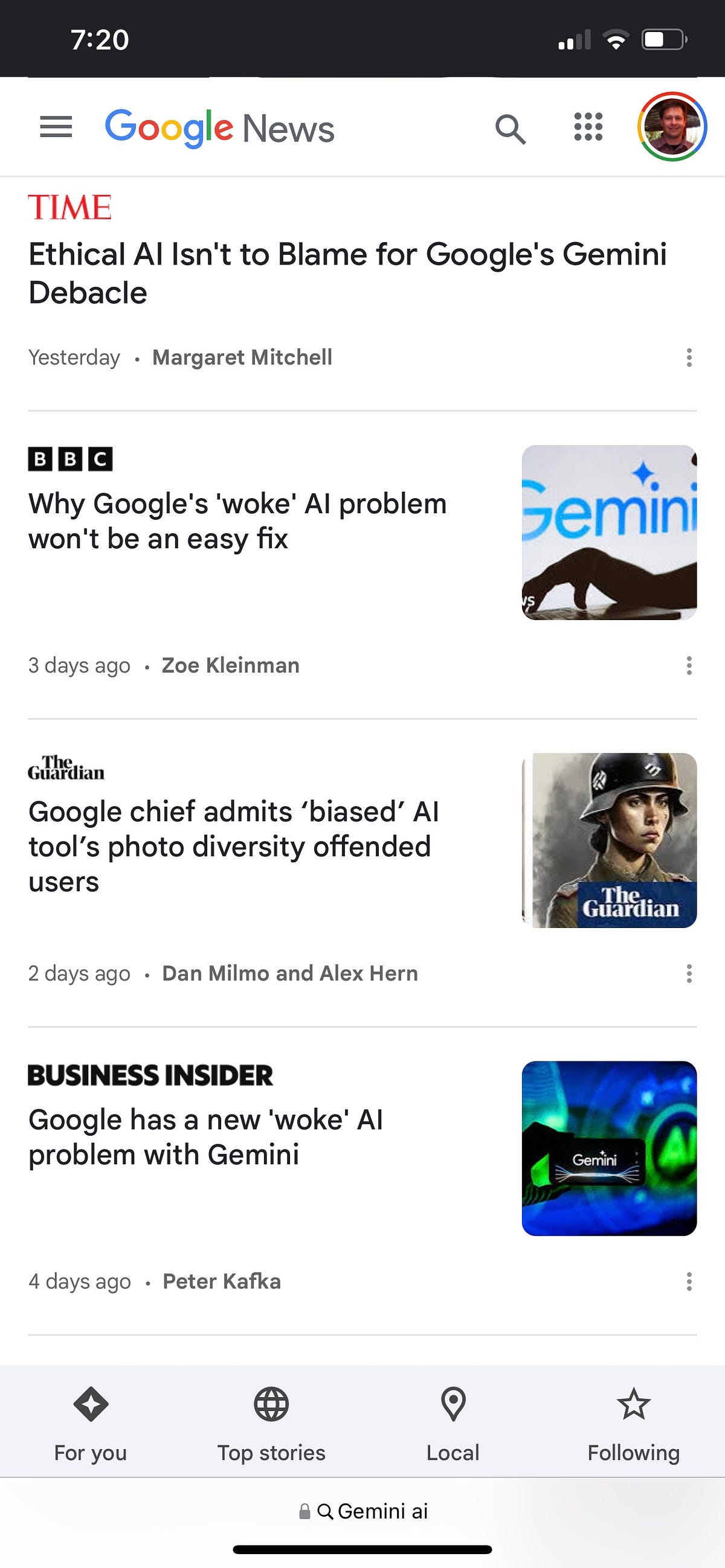The image portrays a Google News interface with several stories listed. At the top of the image, there is a long black bar. On the left side of the bar, the time is displayed in white as "7:20." Below the time, there are three horizontal lines, symbolizing the menu icon. Beside this, the word "Google" appears in its iconic colorful lettering (blue, red, yellow, and green), followed by the word "News."

On the far right side of the black bar, within a Google-like circular icon, there is an image of a man's face. Below this, in red font, the word "Time" is displayed.

Moving down, the main story headline reads: "Ethical AI isn't to blame for Google's Gemini debacle," written in black text. In smaller text below the headline, it says, "Yesterday, Margaret Mitchell," separated by a long line.

The next featured story is indicated by three black squares, each with the 'BBC' logo inside. The headline for this story reads: "Why Google's woke AI problem won't be an easy fix."

Further down, a section from The Guardian highlights an image of a woman wearing a soldier hat. The accompanying headline reads: "Google chief admits 'biased' AI tools photo diversity offended users." 

The final story in the list is from Business Insider, written in all capital letters, stating: "GOOGLE HAS A NEW WOKE AI PROBLEM WITH GEMINI." To the right of this headline, there is a square icon filled with neon green and blue colors.